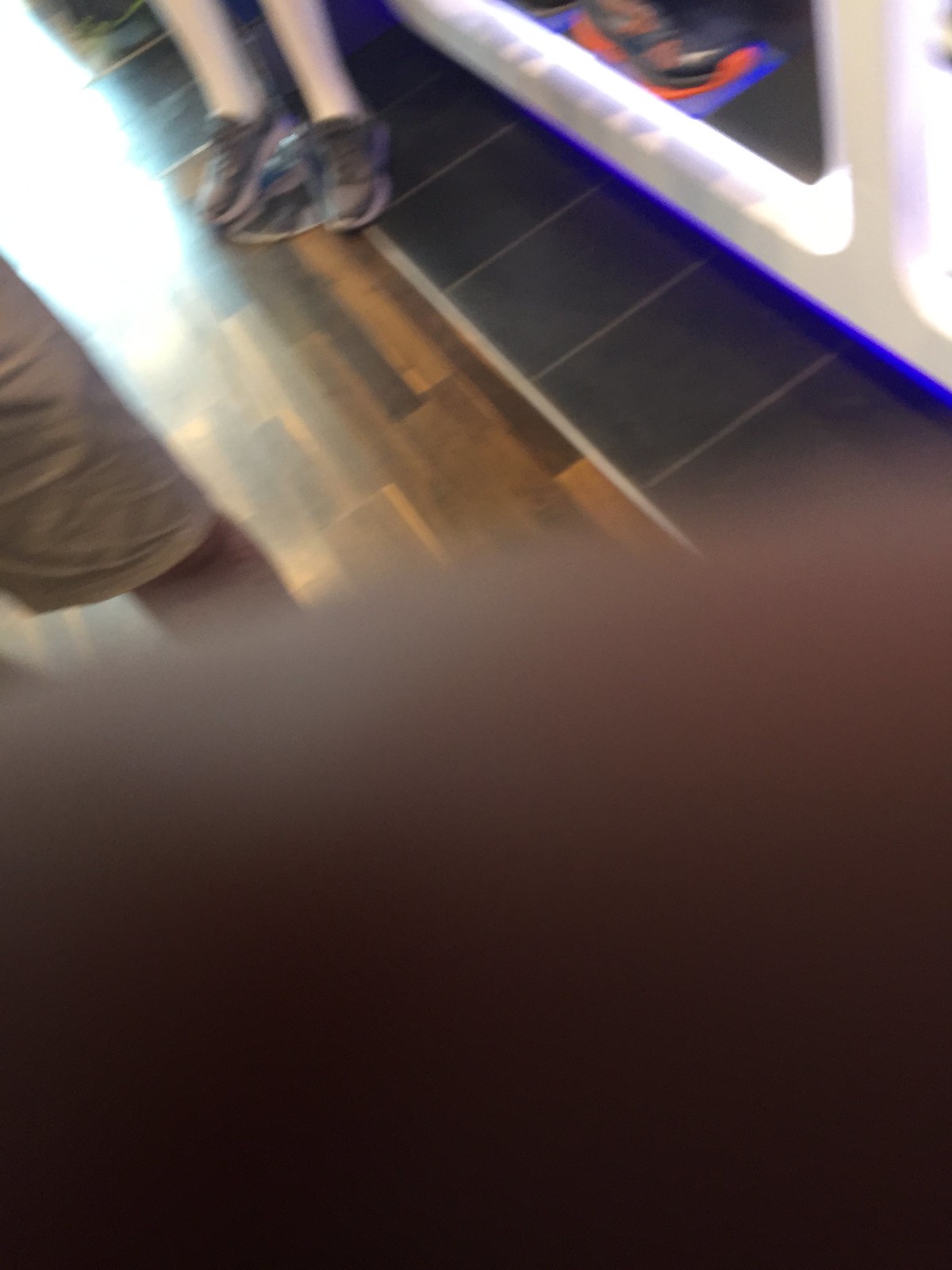This blurred photograph appears to have been taken by accident. It captures an ambiguous scene where various elements are partially visible. The floor is a mix of tile and wood, suggesting a transitional space, perhaps between rooms. On the left side, the lower portion of a pant leg is visible against a white wall. Moving to the right, a pair of black sneakers and pale legs can be seen, indicating someone standing nearby. A bright blue light emits from an unidentified source beside another section of white wall. Beyond this, a pair of brown shoes, likely men's, can be spotted. Dominating the lower half of the image is a large thumbprint, further emphasizing the inadvertent nature of the photo.